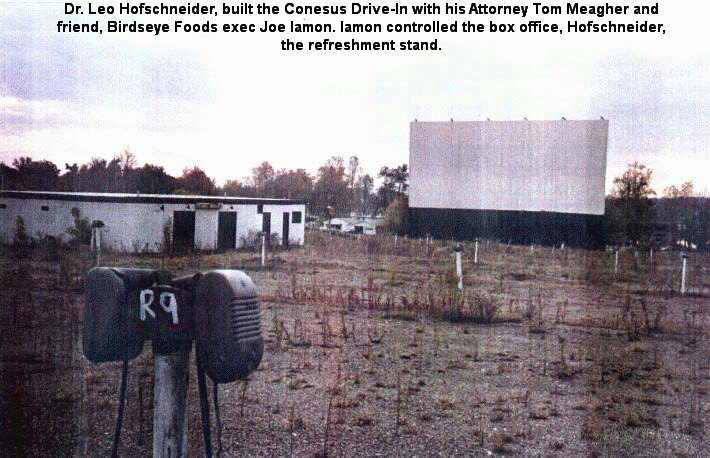This black-and-white photograph captures the hauntingly nostalgic scene of an old abandoned drive-in theater. Dominating the background is a massive, weathered white screen, a silent remnant of bygone days of outdoor cinema. In the foreground to the left stands a pole marked "R9," adorned with twin relic speakers that once broadcast movie audio into car windows. The overgrown parking area is a telltale sign of years of neglect, with grass and weeds sprouting defiantly through the fractured pavement.

At the very top of the image, a faded textual overlay recounts the drive-in's history, reading: "Dr. Leo Hofschneider built the Consensus drive-in with his attorney Tom Meagher and friend, Birdseye Foods exec Joe Lamone. Lamone controlled the box office, Hofschneider the refreshment stand." A humble, white one-story structure with four black doors and without noticeable windows, potentially the refreshment stand, can be seen in the mid-ground, adding to the air of desolation.

The entire scene is drenched in a sepia tone, lending a vintage feel to this poignant snapshot of a once vibrant community entertainment hub, now silently overtaken by time and nature.